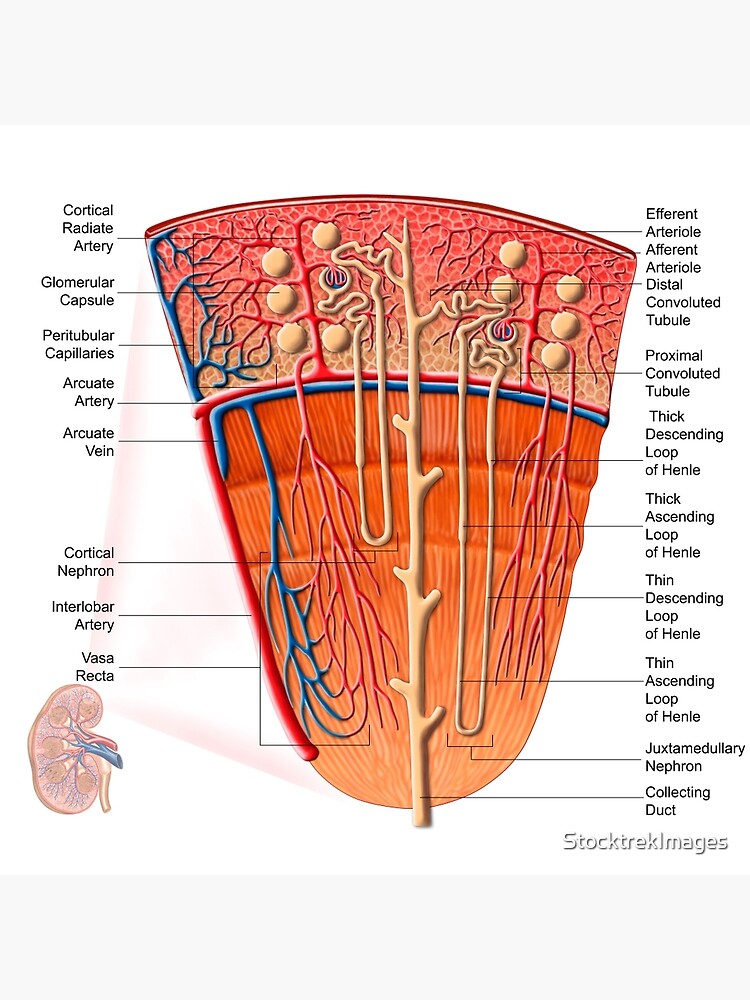The image is a detailed, histological cross-section diagram from a biology or anatomy textbook, depicting a segment of the kidney, particularly focusing on a nephron unit. It vividly illustrates various anatomical components in vibrant colors: arteries are marked in red, veins in blue, and the nephron lumens in a yellowish hue. The top of the diagram is triangular, descending into a curved semicircle at the base. Numerous labels pinpoint specific structures including the cortical radiate artery, glomerular capsule, peritubular capillaries, arcuate artery, arcuate vein, cortical nephron, interlobar artery, vasorecta, afferent arteriole, distal convoluted tubule, proximal convoluted tubule, thick and thin loops of Henle, juxtamedullary nephron, and collecting duct. The left side showcases an intricate network of colored veins and arteries, while the right features a prominent brownish stem with a branching pattern connecting various parts of the nephron unit. Text labels stipulating the aforementioned terms are meticulously placed around the diagram, aiding in identification and understanding of each structure. A watermark stating "duct trek images" is located at the bottom right corner of the image.